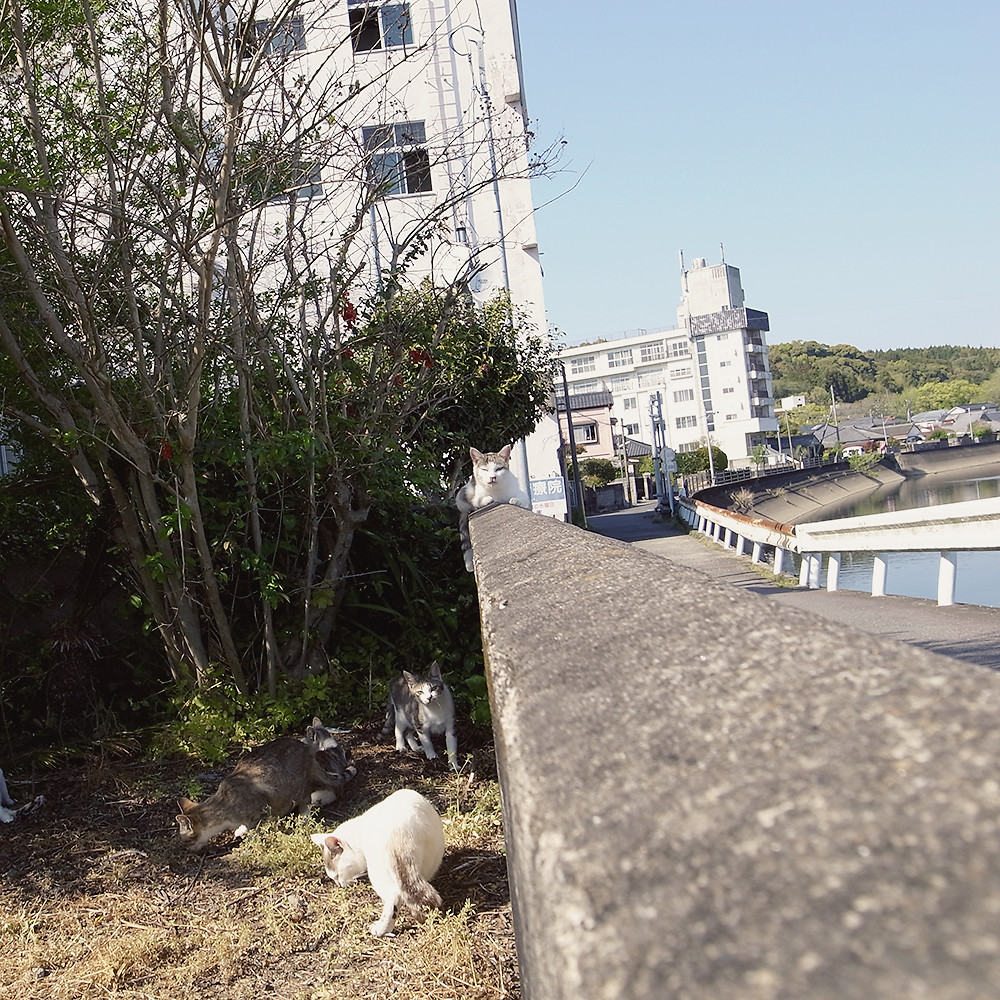The photograph captures an outdoor scene featuring several cats and distinctive architectural elements. Dominating the foreground is a concrete retaining wall that runs horizontally across the image, with a white cat lounging on its belly on the wall's lip, facing the camera with a mix of curiosity and nonchalance, its darker ears and gray tail adding contrast. Below, on the ground near a tree with green and a few red leaves situated towards the lower left, there are three more cats: a white cat roaming around, a striped white cat, and a gray cat in a pouncing position, all engrossed in their activities on the ground.

The background showcases a serene setting with white, multi-story buildings that feature windows and terraces facing the right. The buildings, with one partially obscured behind another, create a layered cityscape. To the right, a low white fence encircles a visible body of water, while signs of rust on its upper rail add a touch of rustic charm. The right side of the image includes a road running parallel to the retaining wall. The lush greenery and branches interspersed throughout the scene, likely from bushes or trees, soften the urban hardness of the concrete and buildings. The well-balanced composition of the photograph merges the tranquility of nature with the quiet companionship of the gathered cats.